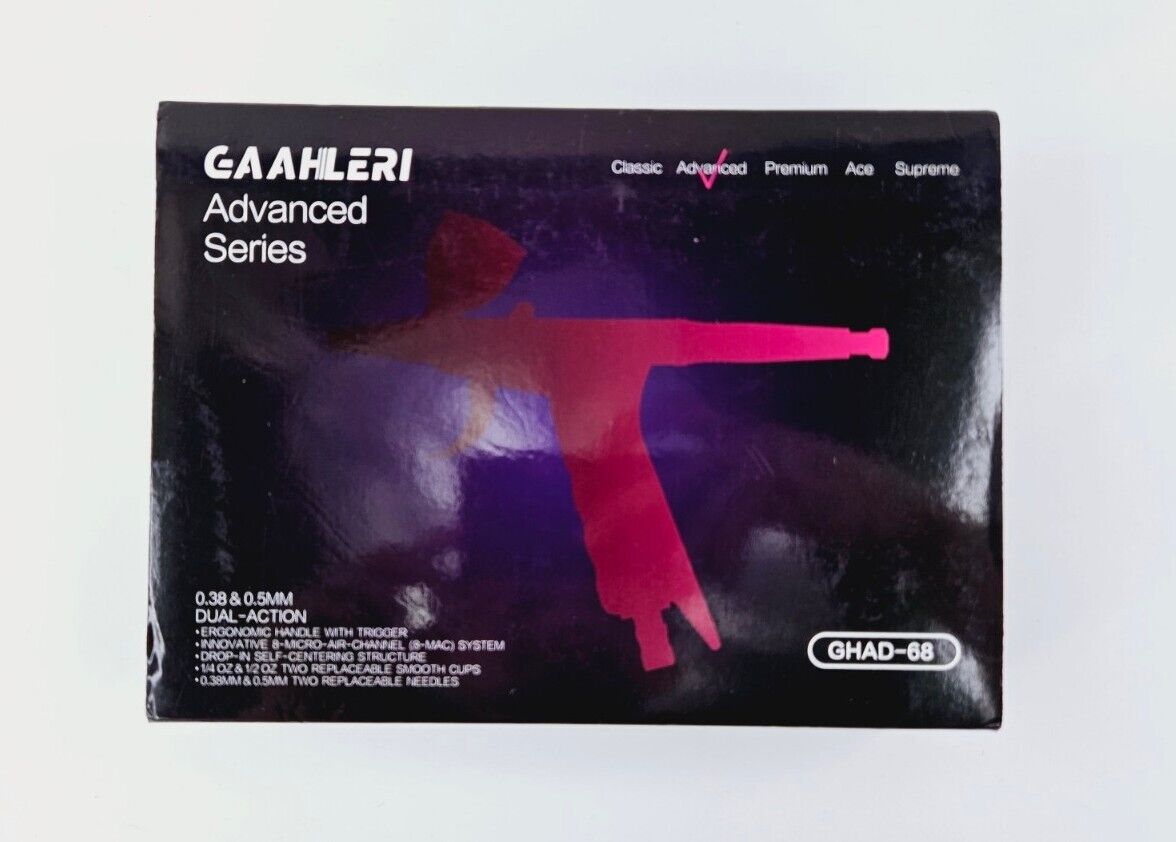The image features a photograph of a package centered against a solid gray background. The package itself is small, square, and appears soft with a slightly longer width than height. Dominating its design is a black background with a vague pink gun illustration in the center. In the upper left corner, the text "Gallery Advanced Series" is prominently displayed. To its right, phrases such as "Classic Advanced Premium Ace Supreme" are listed. The lower right corner features the text "GHAD-68" within a rounded rectangle. On the lower left, there are detailed bullet points describing features such as "0.38 and 0.5 mm dual action ergonomic handle with trigger," "innovative 8 micro air channel," "8 max system," "drop-in self-centering structure," "1/4 oz and 1/2 oz replaceable smooth cups," and "0.38 mm and 0.5 mm replaceable needles," all in white text. This detailed packaging suggests it contains an accessory related to guns, likely focusing on precision and ergonomic design.